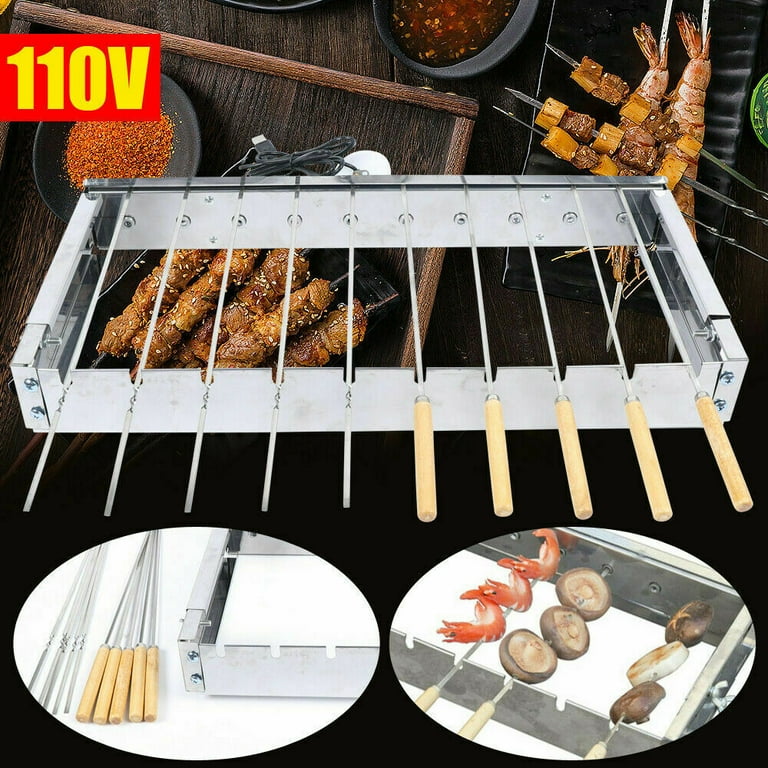The image depicts an advertisement for a rectangular kebab grill assembly specifically designed for making shish kebabs. The grill is centrally showcased with ten skewers aligned across it—five on the left side without handles and five on the right with wooden handles. Above the image, in a yellow text surrounded by a red box, it indicates "110V." 

The background vividly illustrates various cooked shish kebabs, featuring square pieces of meat, large prawns, potatoes, corn, lobsters, and a medley of vegetables, all seasoned with different spices visible in three bowls at the top. 

At the bottom of the image, two oblong circles provide further details. The left circle highlights the skewers alone, differentiating between the plain metal skewers and those with wooden handles. The right circle displays three skewers loaded with food: one with shrimp, one with mushrooms, and the third with an assortment of vegetables and more mushrooms.

Overall, the advertisement emphasizes the versatility and functionality of the grill for an array of ingredients, complete with a clear demonstration of its components and usage.